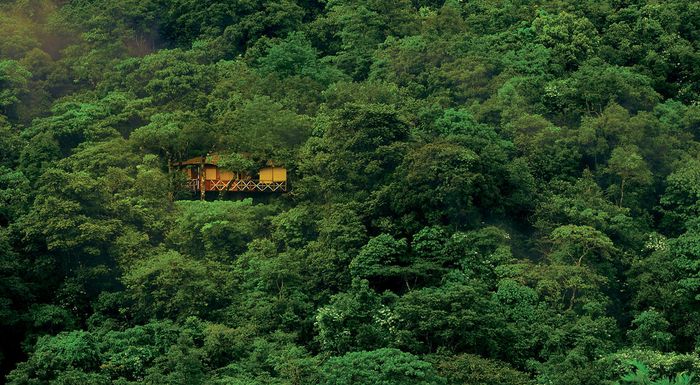The photograph captures a quaint one-story house nestled amidst a densely wooded hillside, taken from a vantage point on an adjacent hill. The house, predominantly yellowish-golden with brown detailing and a brown roof, is situated slightly to the left and towards the middle of the image. Much of its roof is obscured by the surrounding trees, some of which extend onto the roof itself. The dense forest of rich, dark green leaves fills the entire frame, with an almost uniform hue. The lower left corner marks the base of the hill, ascending to the upper right, where the hill peaks. The upper left corner of the photo is slightly blurry, hinting at the presence of some brownish trees. The scene is brightly lit by natural daylight, underscoring the clarity and vividness of this serene outdoor setting.